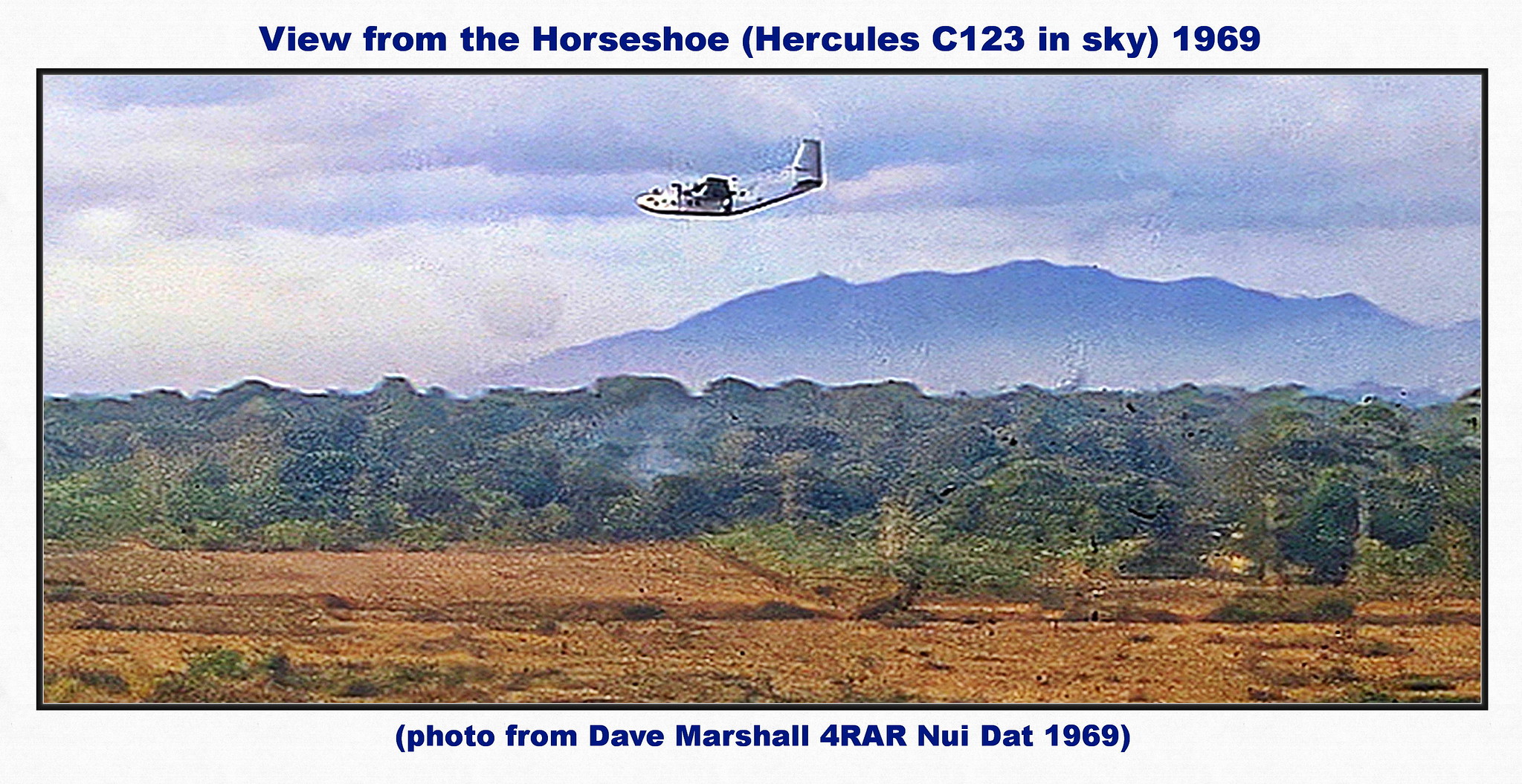The image is a horizontally aligned rectangular photograph against a light gray background, with a black border framing it. The scene captures a Hercules C-123 aircraft, predominantly white and black, flying towards the left. The image, dated 1969, appears grainy and of lower quality, typical of the period.

The sky is overcast with a mix of purplish-blue and white clouds. Below the aircraft, towards the horizon, there's an outline of mountains or hills. In the midground, a dense forest of green trees is visible. The immediate foreground features a flat, brown area that could either be dead grass or dirt, resembling an improvised airfield.

Text at the top of the image in dark blue reads: "View from the Horseshoe" with "(Hercules C-123 in sky)" and "1969" in parentheses. At the bottom, another caption in parentheses states: "Photo from Dave Marshall, 4RAR NUI DAT, 1969."

This photograph offers a historical glimpse into the skies of Vietnam during the era, showcasing a significant cargo aircraft amidst a landscape of clouds, mountains, and trees.